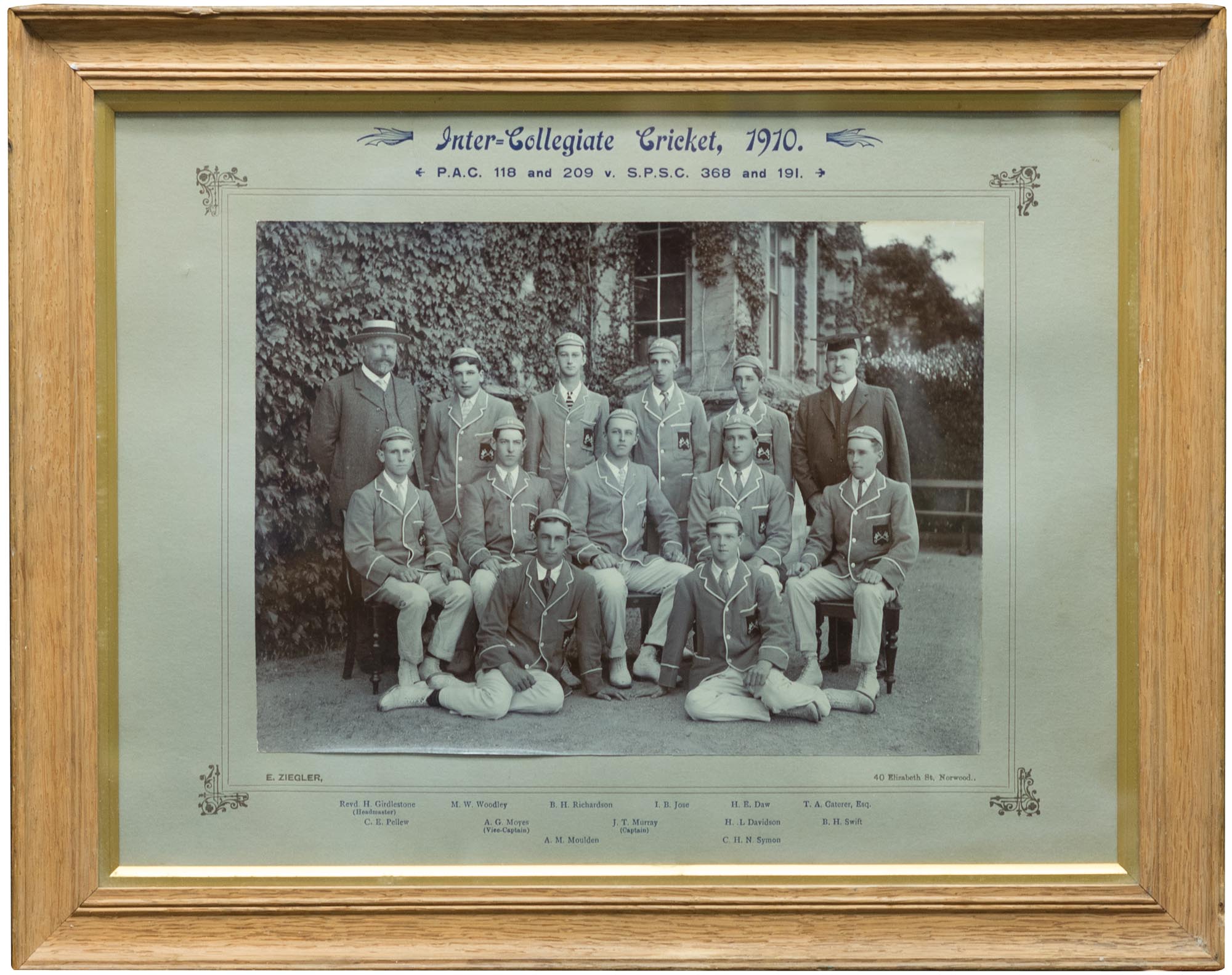This black-and-white photograph, framed in a pine-colored wooden frame, captures a historic intercollegiate cricket team from 1910. The image features thirteen men in total, consisting of eleven players and two coaches. The team members stand and sit uniformly dressed in suits with ties, light pants, and shoes, paired with darker jackets. The two coaches are positioned at each end of the group; the coach on the left sports a wide-brimmed hat, while the one on the right wears a dark graduation cap. The photograph was taken outdoors in front of a building adorned with vines, with six men standing, five seated on chairs, and two seated on the ground. Each individual in the picture appears content, and the bottom of the photo includes the inscription: "Intercollegiate Cricket 1910, PAC 118 and 209 vs SPSC 368 and 191," along with the names of the team members. The photo is attributed to the photographer E. Ziegler.